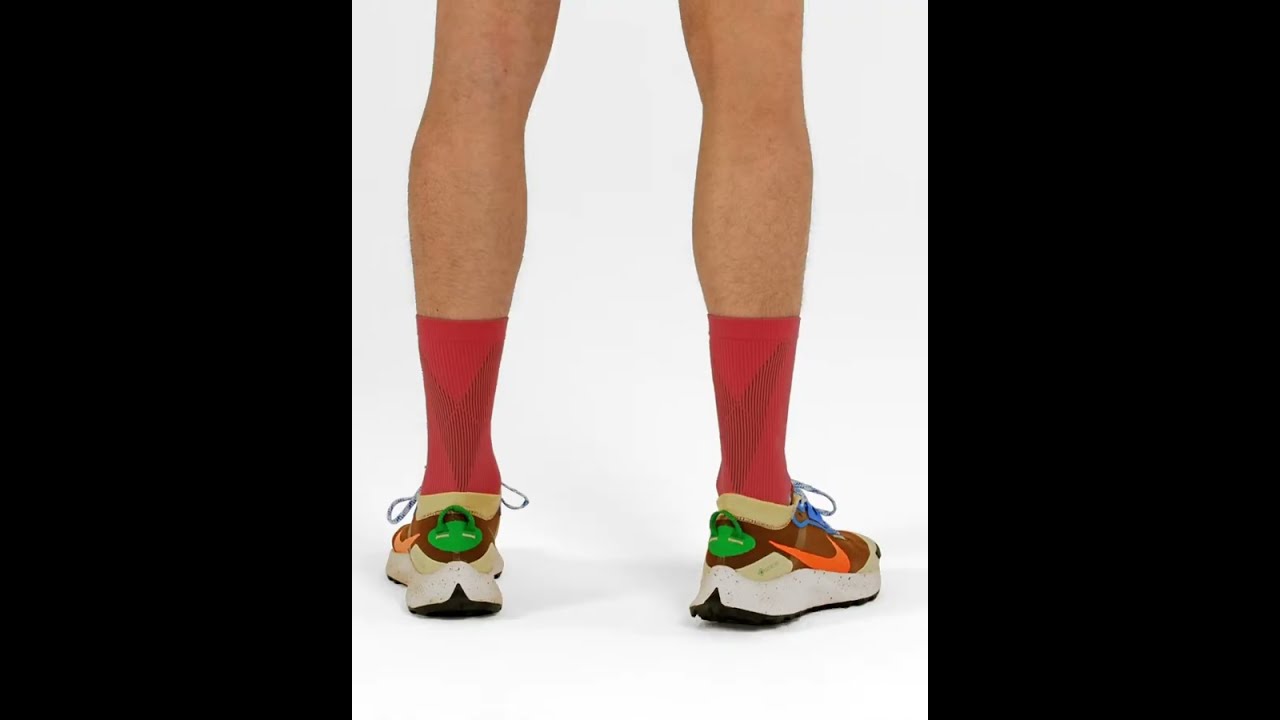The image features the lower half of a person’s legs, from just above the knees down to the feet, set against a pure white or transparent background. The legs are pale-skinned and unclothed until they reach calf-length, tightly fitted red socks that feature a black logo on the back. The person is wearing Nike athletic shoes which are prominently detailed with brown uppers, a distinctive orange Nike swoosh, and bright blue laces. The soles of the shoes are thick and white, with black on the bottoms. A bright green loop is present at the back of each shoe, aiding in their removal. The image is centered with black rectangles on either side, transforming the vertical photo into a landscape orientation, and the person’s heels are facing toward the camera.